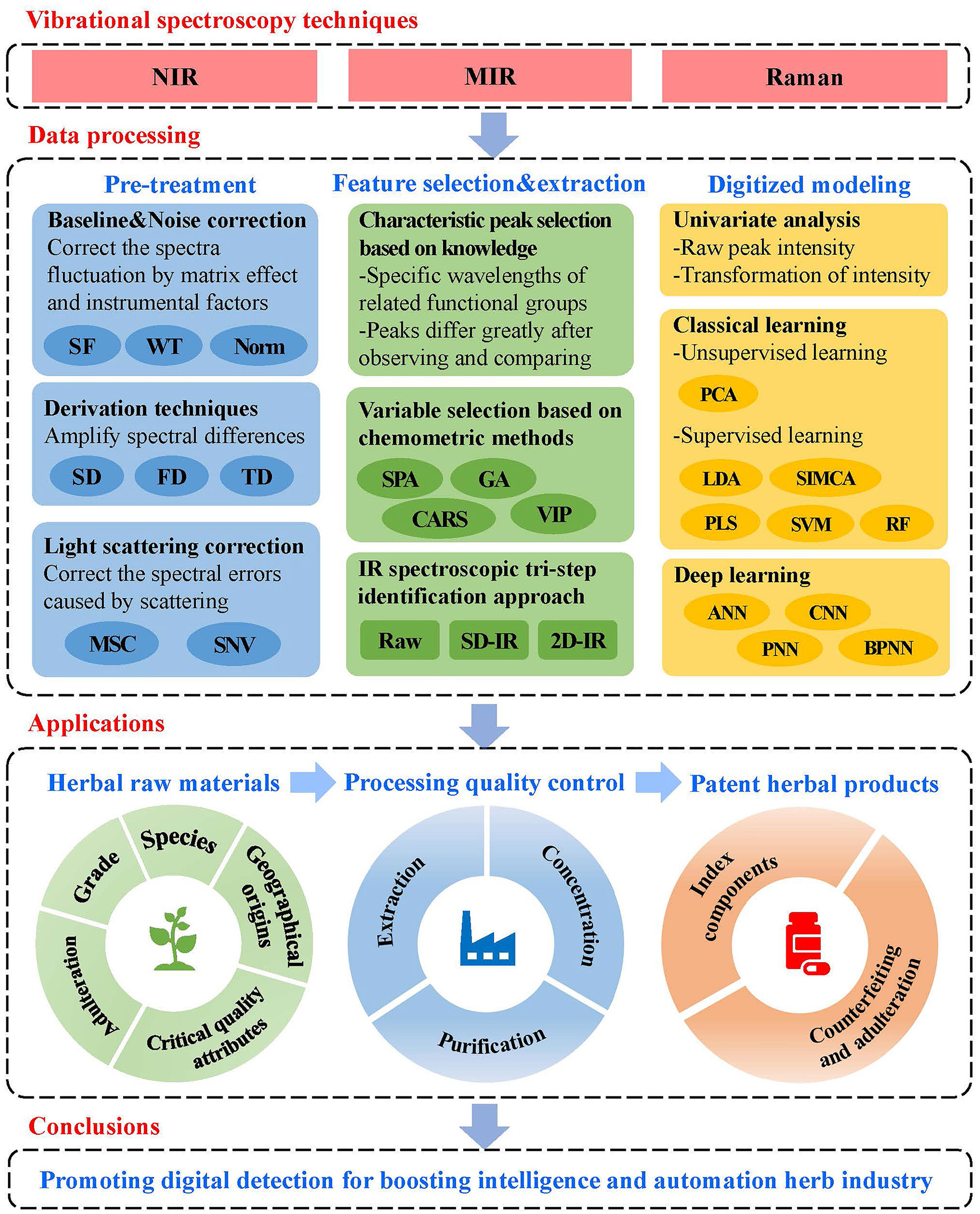The image is a detailed diagram of vibrational spectroscopy techniques, prominently titled in red letters. It includes step-by-step data processing instructions with sections in different colors: blue for pre-treatment (covering baseline and noise correction, duration techniques, and light scattering correction), green for feature selection and extraction, and yellow for digitalized modeling. Key spectroscopy types such as NIR, MIR, and RAMAN are highlighted, with checkered grayish-black lines indicating their connection to subsequent data processing steps. 

Blue arrows point downward to illustrate the flow of information through various stages, leading to applications in herbal raw material processing, quality control, and patent herbal products. At the bottom, informational wheels shaped like donuts encircle terms related to these applications, emphasizing their significance in the process. The diagram concludes with text that promotes "digital detection for boosting intelligence in the automation herb industry," highlighting the practical and modern applications of these techniques. The style and layout resemble an instructional manual, using a variety of colors—red, blue, green, yellow, and tan—to differentiate the sections and enhance clarity.